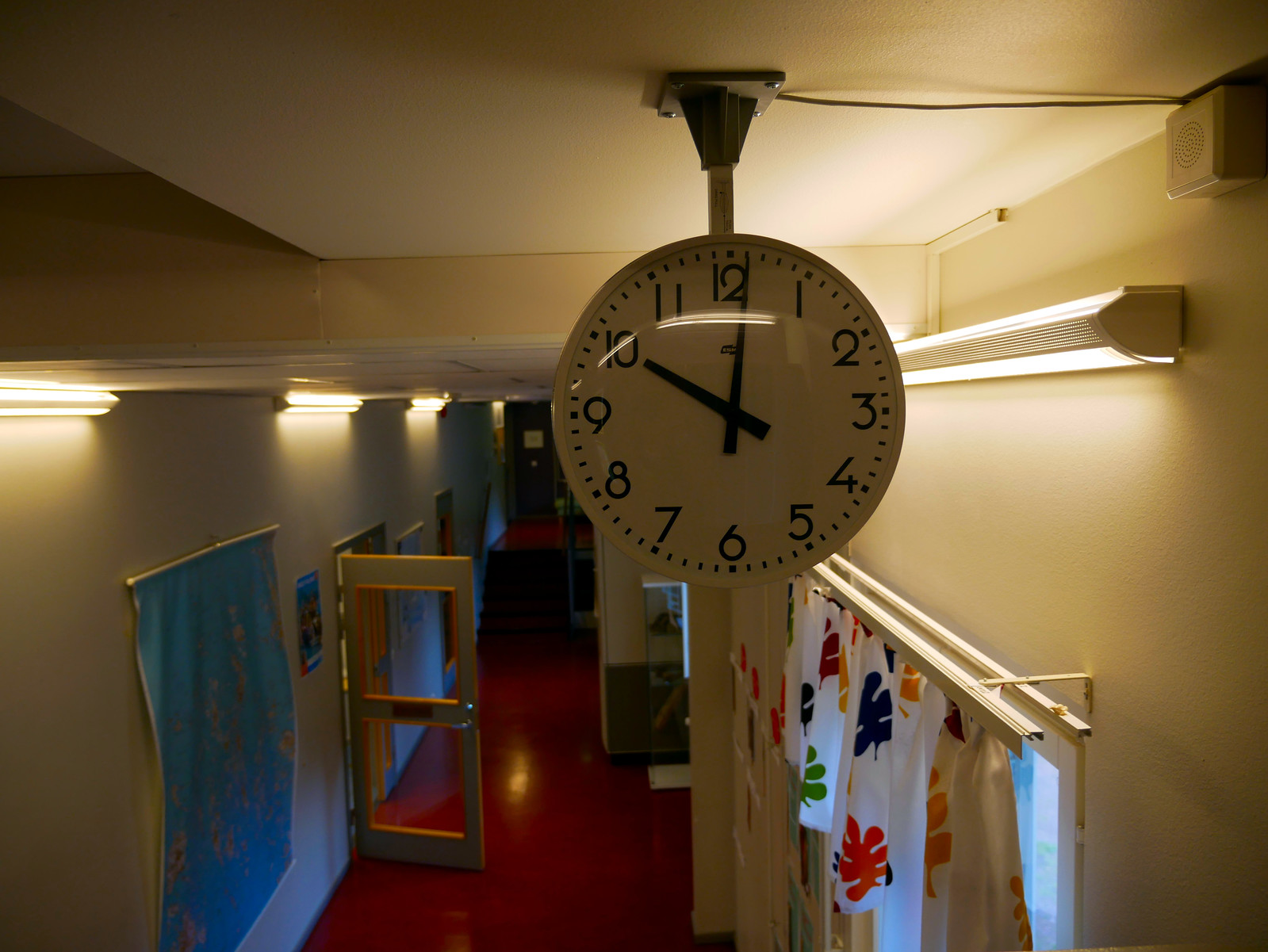This photograph captures a clock suspended from the ceiling in what appears to be a school hallway. The ceiling and walls are painted a soothing cream color, providing a calm backdrop. The clock, featuring a minimalist design with a white face, black numerals, and matching hands, is encased in glass—a detail highlighted by the reflection of overhead lights. It is mounted on a robust, gunmetal silver bracket fastened securely to the ceiling.

Directly beneath the clock, a window adorned with a short, white curtain comes into view. This curtain is accentuated with a vibrant leaf pattern in red, blue, green, and yellow, adding a touch of color and cheerfulness. On the opposite wall, a large, detailed map is prominently displayed. 

The floor below is a striking bright red, its glossy, pristine finish suggesting highly polished linoleum. Nearby, a wooden door featuring a glass panel both at the top and bottom stands ajar, hinting at the possibility that it leads into a classroom. Overall, the setting undeniably suggests the hallway of an educational institution.